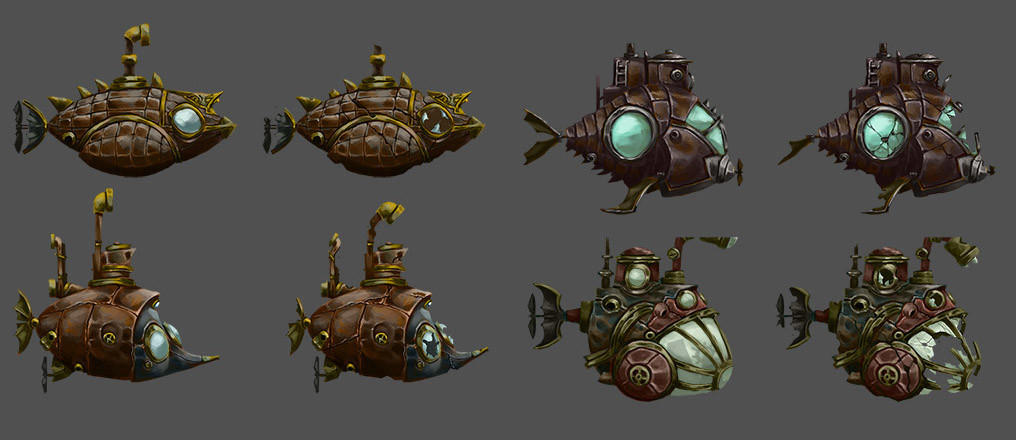The image is a horizontal gray rectangle displaying eight cartoon-style underwater vehicles, resembling submarines designed to look like different types of fish. The submarines appear in two rows of four, with the top row featuring side views of primarily dark brown submarines with light green windows, and various distinguishing features: 

- The first submarine has a clear, round window at the front resembling an eye, a periscope extending from the middle, and a fin on the back mimicking a fish's tail. 
- The second submarine is similar, but with a broken front window showing shards of glass.
- The third submarine is darker and at an angle, with front windows of different shapes, a periscope missing, and a different fin configuration.
- The fourth submarine is similar to the first, but has a broken side window and a partially broken back fin.

The bottom row mirrors the top row with variations in the front windows, periscopes, and back fins, exhibiting different stages of damage or alternate designs. The overall image appears to be concept art for mechanical fish-like submarines, standing out clearly against the dark gray background.